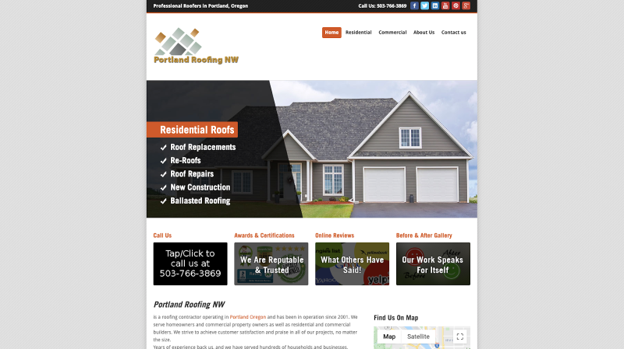The image depicts a comprehensive layout of a professional realtor’s website based in Portland, Oregon. The backdrop is primarily light gray, while the main content window features a white background complemented by a black header with bold white lettering that reads, "Professional Realtors in Portland, Oregon." On the right side of the header, a call-to-action message, "Call Us:" is prominently displayed alongside a listed phone number.

Below the header, there is a white banner with gold accents on the left, displaying the text, "Portland Roofing NW," alongside images of gray roofing panels. The center panel is a darker shade of gray than the others. Additionally, there are two gold squares situated in the upper left and right corners of this section.

To the upper right, the main navigation menu is prominently visible. The currently selected menu item, "Home," is highlighted in bold white text set against an orange background. The other menu options—"Residential," "Commercial," "About Us," and "Contact Us"—are displayed against a white background with bold black text.

The central image captures a picturesque residential setting under a vivid blue sky. A grayish-beige house with a two-door garage and a two-panel window above the garage is featured prominently. The roof of the house is covered with gray shingles. On the left side of the image, there is a slanted, transparent black overlay. Overlaying this section, a label with an orange background and bold white lettering reads, "Residential Roofs." Below the label, a checklist itemizes the services offered, each marked with a white check. The services listed are: "Roof Replacements," "Re-roofs," "Roof Repairs," "New Construction," and "Balustrade Roofing."